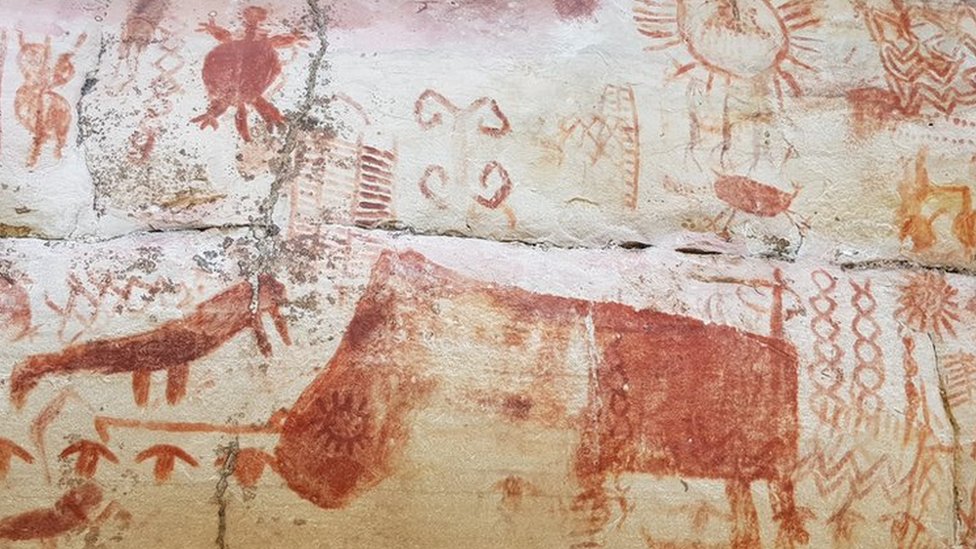The image showcases what appears to be ancient or abstract cave paintings on a crackly and uneven white surface, possibly wood. Dominating the scene is a large reddish animal with a broad muzzle, likely a moose or similar creature, situated at the bottom center and facing left. Surrounding this central figure are several other indistinct animals and designs predominantly in shades of red, with some yellow accents. In the top left quadrant, a red turtle heads upward, while a bright sun and a crab are visible towards the right. The bottom left section features a series of eyes, including visible pupils and eyebrows, adding to the mysterious imagery. On the bottom right, circular designs and triangular shapes can be seen, alongside a figure that resembles a person with horn-like features. The artwork, which lacks detailed brushwork, suggests that finger painting might have been used, further adding to its primitive and intriguing appearance.